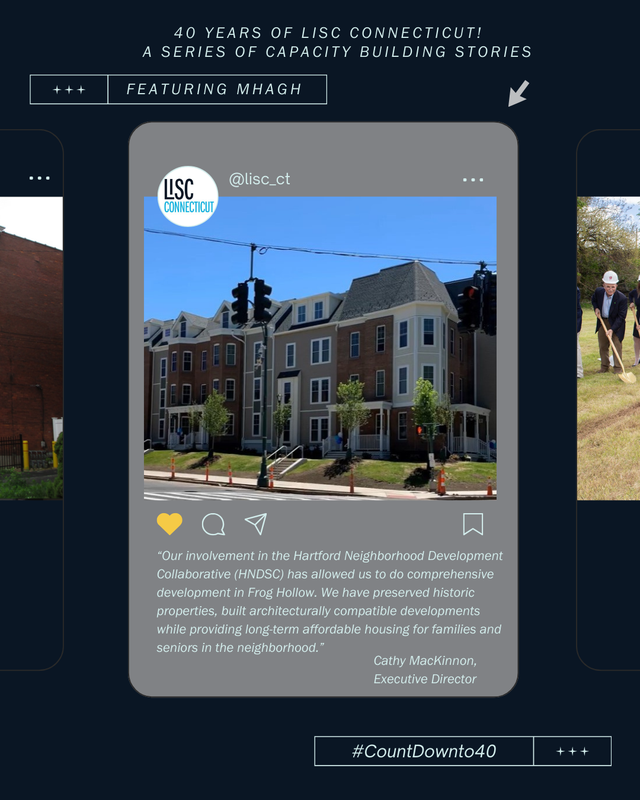Celebrating 40 years of LISC Connecticut: A series spotlighting capacity-building stories featuring MHOG and USLICS. Our collaboration with the Hartford Neighborhood Development Collaboration has enabled significant work in Frog Hollow, including the preservation of historic buildings and the involvement of architecturally compatible developers, among other achievements. Countdown to 40 years of impact! #40YearsOfLISC 💛➡️